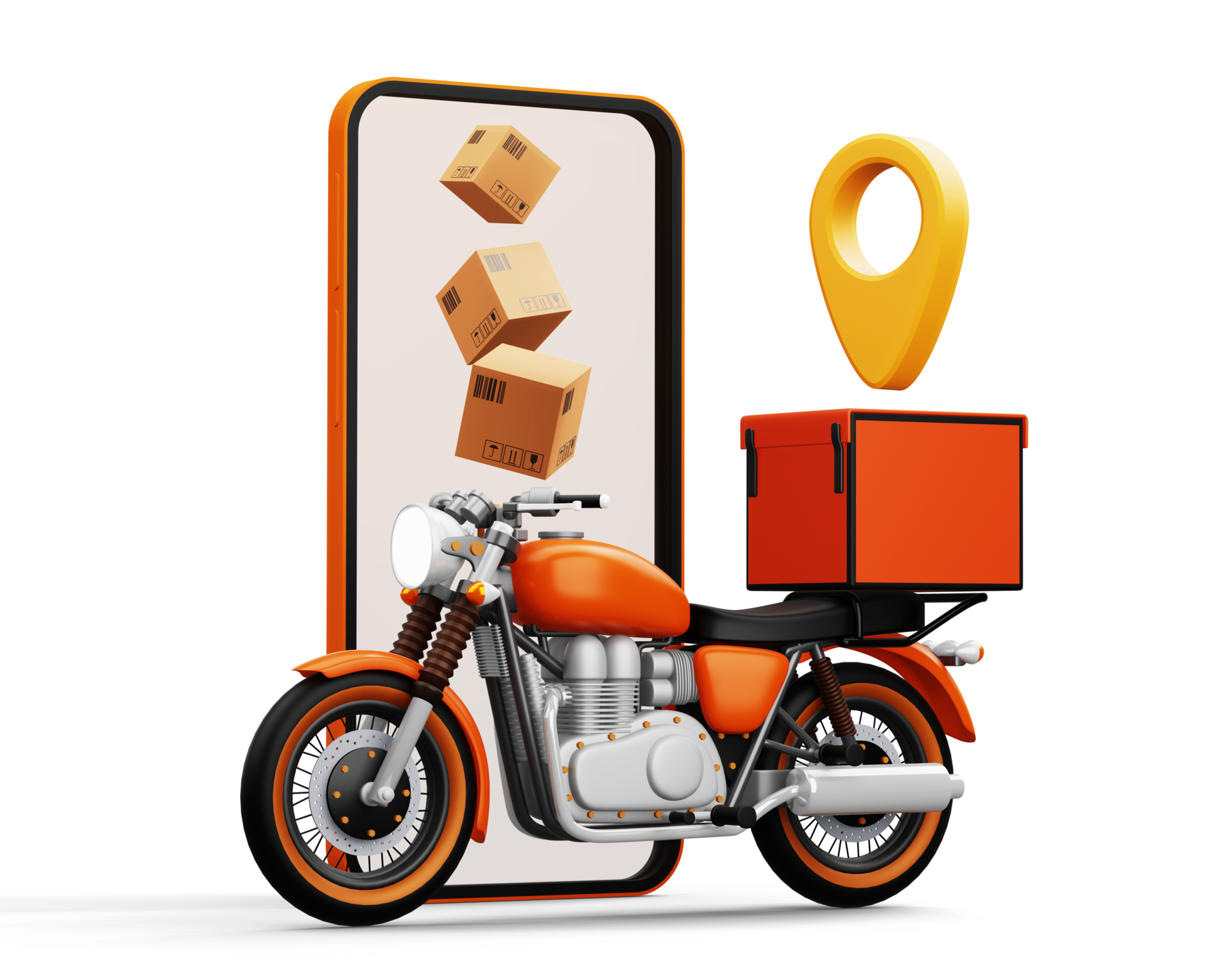The image depicts a whimsical, cartoonish orange motorcycle positioned in front of a smartphone. The motorcycle features a predominantly orange color scheme, with an orange gas tank, wheel wells, and tire liners, complemented by a black leather seat, a metal gray side, and a chrome muffler. At the rear of the motorcycle sits a large orange delivery box, above which hovers a yellow map pin icon with an inverted teardrop shape and a hole through the top. The smartphone behind the motorcycle, encased in orange, prominently displays three cardboard boxes with barcodes and shipping symbols tumbling down the screen. The overall setting suggests a playful and vibrant theme, perhaps alluding to fast delivery or a new service related to quick shipments.